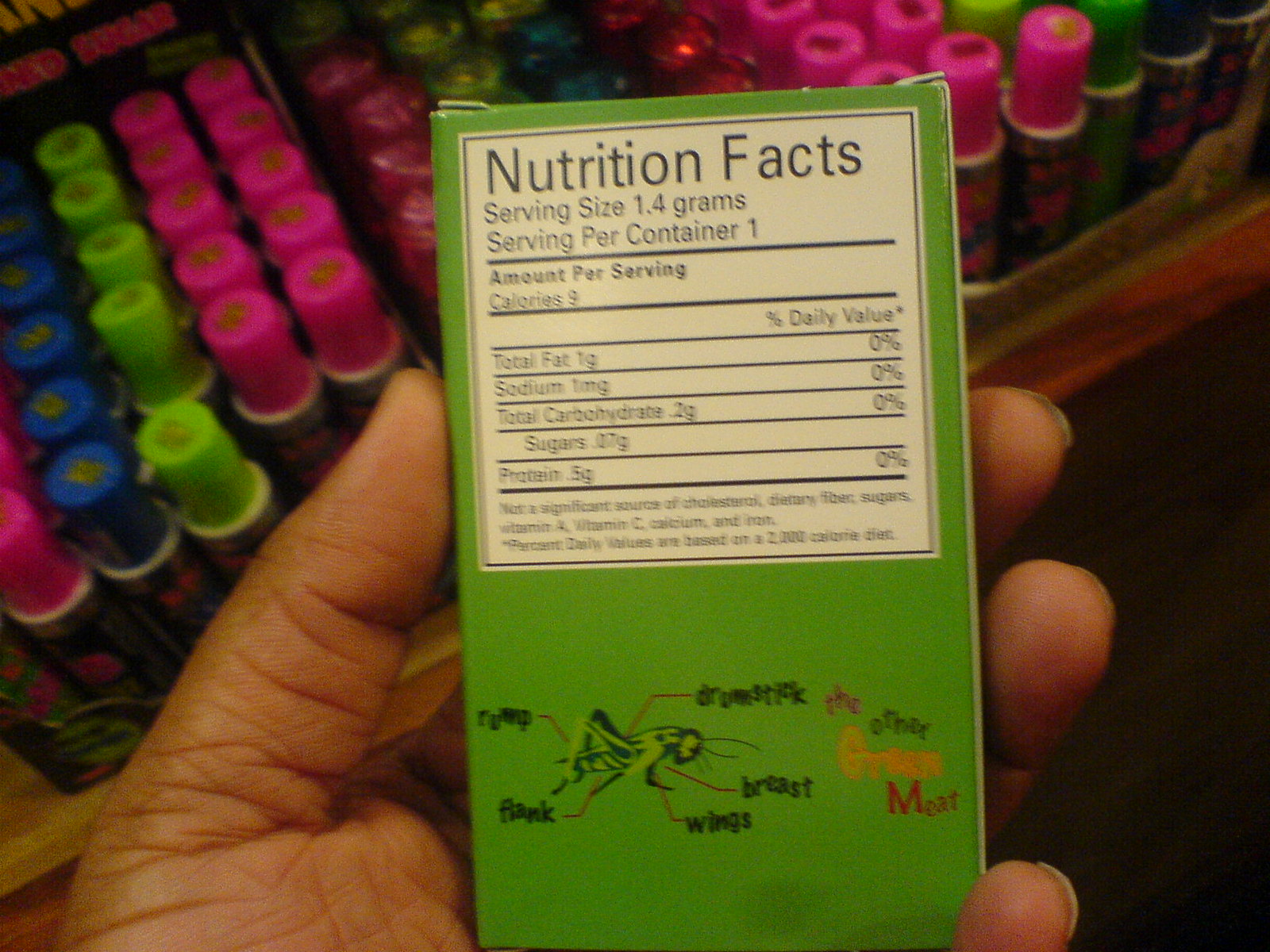In the image, a person's left hand is holding a rectangular green cardboard box, centered in the frame. The box is held in front of a shelf stocked with various products, including items with neon pink, green, lime, and blue tops. The focus is on the white and black nutrition label located at the top of the box. Although slightly blurry, the label reads: "Nutrition Facts. Serving size 1.4 grams. Servings per container 1. Calories 9. Total Fat 1g. Sodium 1mg. Total Carbohydrate 2g. Sugars 0.07g. Protein 5g. Not a significant source of cholesterol, dietary fiber, sugars, vitamin A, vitamin C, calcium, and iron. Percent daily values are based on a 2,000 calorie diet." Below the label, there is an illustration of a grasshopper with labeled body parts: drumstick, rump, flank, wings, and breast, indicating portions like a meat diagram. The box is identified as containing "the other green meat," suggesting it is a novelty or niche food product likely found on a store shelf.